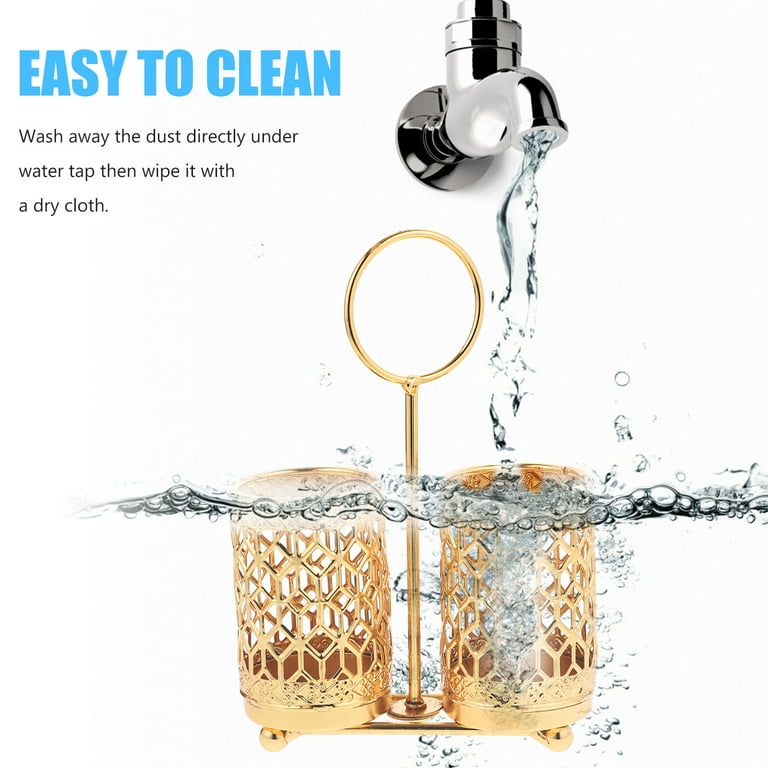A digital, full-color, square photograph features a silver water spigot at the top, positioned against a solid white background with no border. In the upper left corner, bold blue uppercase text reads "EASY TO CLEAN," followed by smaller left-aligned black text that instructs, "wash away the dust directly under water tap then wipe it with a dry cloth." Water pours from the spigot, forming visible streams that cascade downwards towards two intricately designed gold vented cups positioned below. These cups rest on a flat gold base and are connected by a gold rod with a circular handle at the tip. Water splashes are evident around the cups, particularly into the one on the right and in front of the cups, highlighting the text's cleaning demonstration.